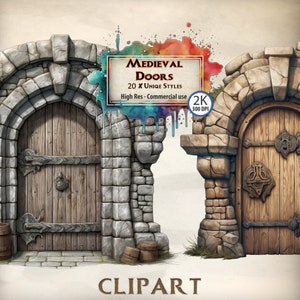The image features detailed illustrations of two medieval-style doors, set against a white backdrop. The door on the left is light gray, framed by similarly colored rocks forming an arch. It features gray bars across the top and a dark brown door handle. In contrast, the door on the right is a lighter brown and framed by light brown stones. This door includes brown bars and a large, somewhat decorative brown spot where the door knob would be. Both doors exhibit intricate details with iron and black metal elements integrated into the design.

Between the two doors, there is a square that says "Medieval Doors," followed by "20 settlers." Below this, there's a circle with "2K" inside, overlaid on a blot of paint with orange and teal hues. At the bottom center of the image, between where the two doors meet, the word "Clipart" is displayed in larger brown lettering. Despite some text being indistinct and compressed, it's clear that the image is promoting a high-resolution, commercial-use clipart pack.